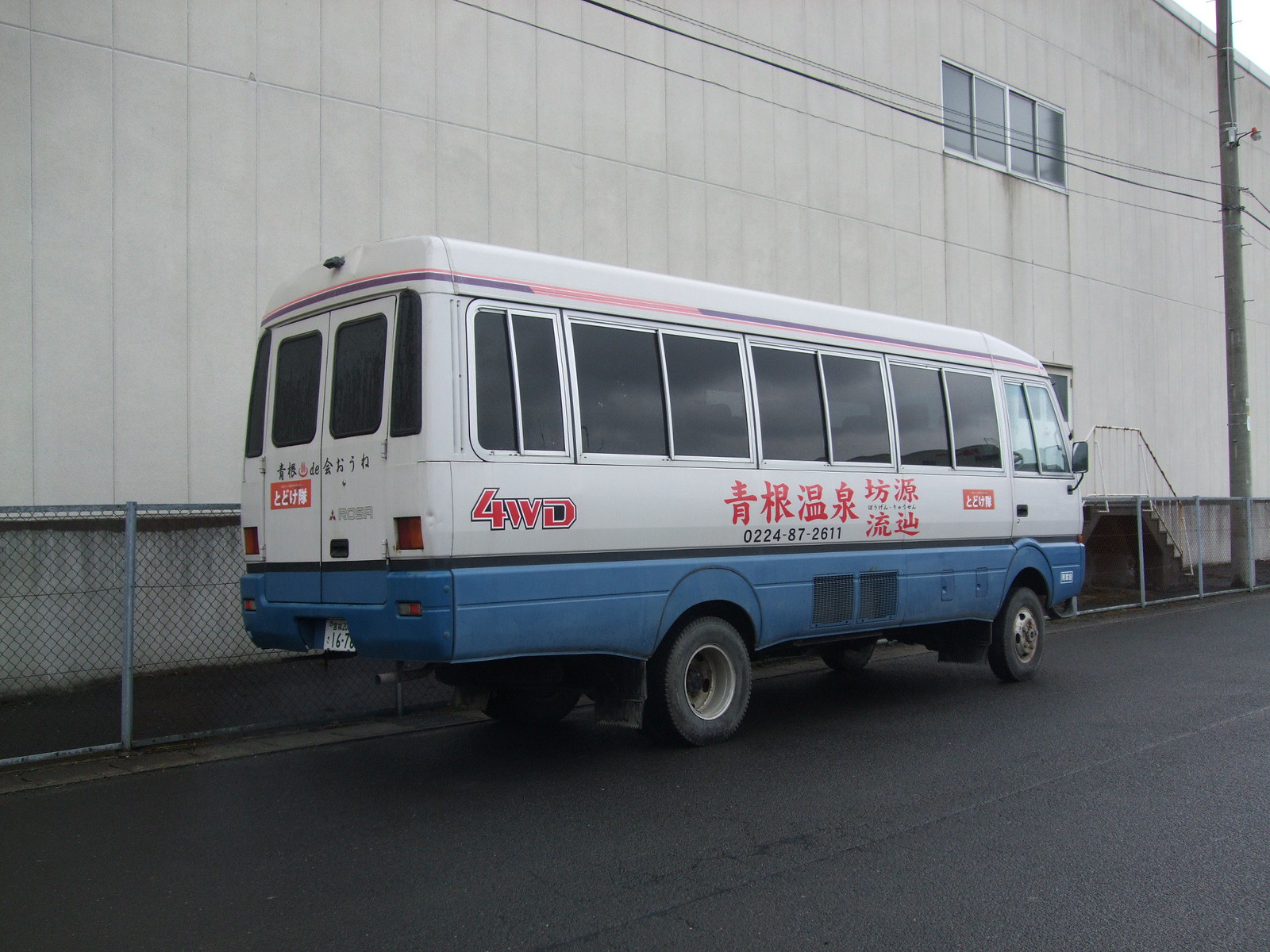The photograph showcases a relatively long van, possibly a mini bus, parked on a black paved road beside a large building, likely a warehouse, with a chain link fence running along its wall. The van stands out with its distinctive design: the lower part is painted blue with a small black stripe, while the majority—approximately 80%—is white. Adding to its colorful appearance, there is also a pink and purple stripe near the top. Notably, the van features dark tinted windows running along both sides and the back. 

The right side and rear doors of the van are adorned with red and black text, presumably in Chinese or another Asian language. A prominent label "4WD" suggests it has four-wheel drive capabilities, and the name "Rosa" can be seen alongside a symbol on the back. The van also displays a phone number, "0224872611," in the red lettering. A small portion of the license plate reveals the numbers "167." The setting includes a visible pole and a building with a singular window, reinforcing the industrial ambiance. A side mirror and details like the tinted windows and black wheels further accentuate the van's robust and practical design.